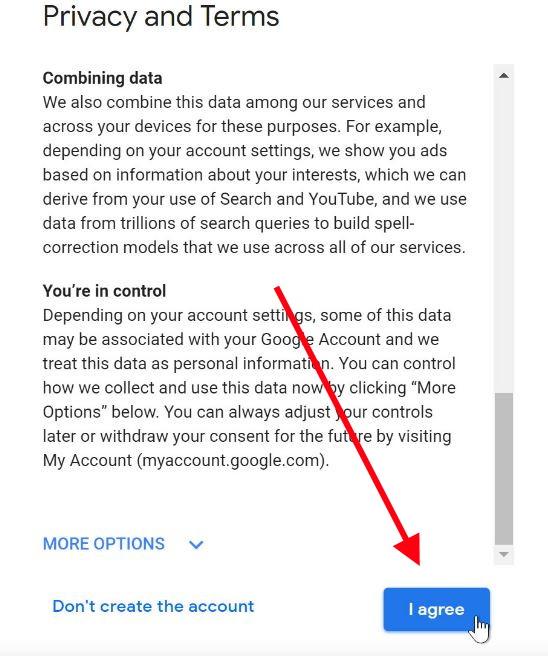A detailed screenshot showing a company’s privacy and data usage policy. It appears to be taken from a computer screen, though this is not definitively clear as there are no indicators like an "X" button to confirm it's a phone interface. The headline "Privacy and Terms" is prominently displayed in large font. 

Below, in bold but smaller font, the section titled "Combining Data" describes how data is aggregated across services and devices. It states: "We also combine this data among our services and across your devices for these purposes. For example, depending on your account settings, we show you ads based on information about your interests, which we can derive from your use of search and YouTube. We also use data from trillions of search queries to build self-correction models that we use across all of our services."

In another bolded section titled "You're in Control," it is explained that: "Depending on your account settings, some of this data may be associated with your Google account, and we treat this data as personal information. You can control how we collect and use this data now by clicking 'More options' below. You can also adjust your controls later on or withdraw your consent for future uses by visiting 'My Account' (myaccount.google.com).”

The options "More options" and "Don't create this account" are displayed in blue font. A red computer-drawn arrow points to the "I agree" button, with a hand-clicking icon hovering over it.